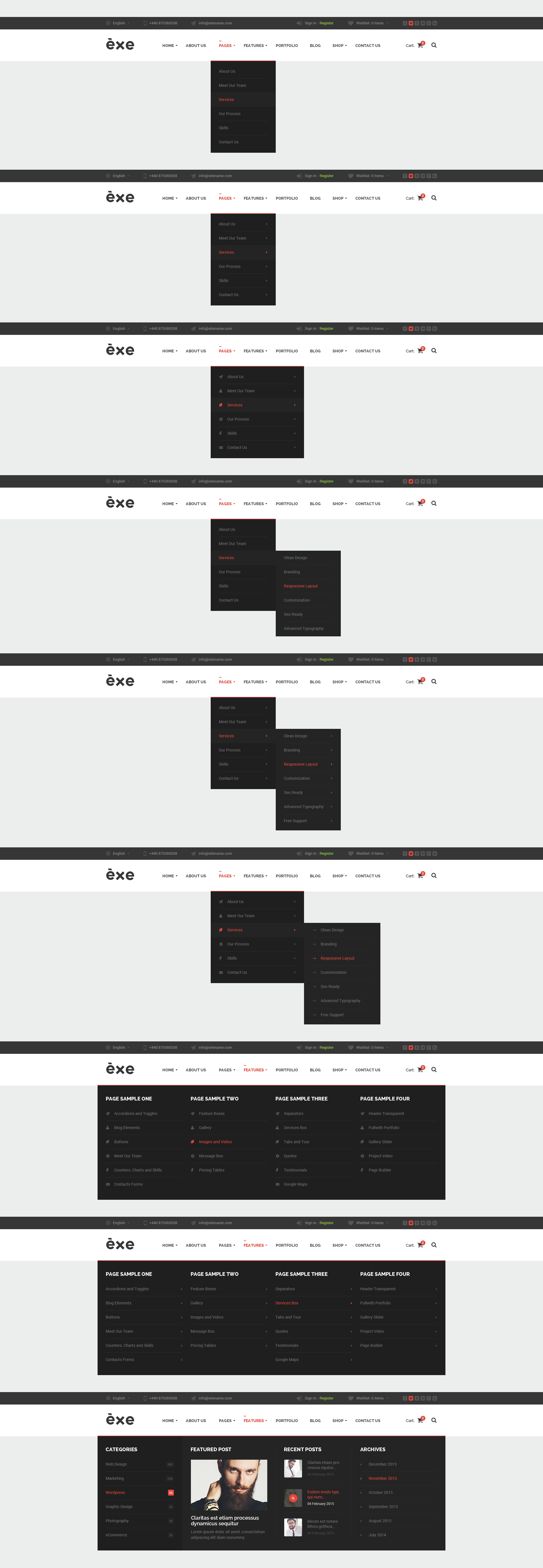The image consists of several horizontally aligned elements against a plain background. At the top, there is a long black bar followed by a long gray rectangle directly below it. Centered within the gray rectangle is a black square. A similar structure repeats in the subsequent row.

The next set of rows shows a variation where the black square is slightly elongated. Following this, there are two rows each featuring two black squares side by side. Progressing further down, one row has a black rectangle connected to a larger black square. This pattern continues with the next row containing a long black rectangle, approximately four inches in length.

In the final section at the bottom, there is another long black rectangle. However, this rectangle includes a small, up-close picture of a man's face. The man's facial features are barely discernible, but it is evident that he has facial hair and fair skin. This image is the only distinguishable visual detail within the otherwise uniform horizontal bars.